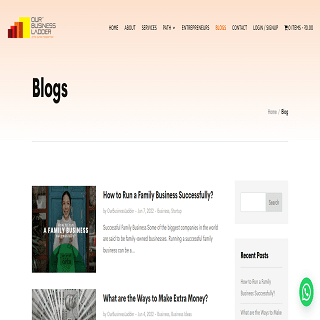The image showcases a section of a website named "Our Business Ladder." In the top left corner, the site’s logo and title are prominently displayed. On the right-hand side of the screen, a navigation menu includes headings such as Home, About, Services, Pay, Entrepreneurs, Blogs, Contact, and Login Group, all set against a light orange background.

Below the navigation menu, the word "Blogs" is featured in a larger black font. A fine grey line runs horizontally across the screen beneath this heading, followed by a series of blog articles. One highlighted article is titled "How to Run a Family Business Successfully," accompanied by a brief description and an image to its left. Another blog entry, "What Are the Ways to Make Extra Money," is similarly presented with additional text and an accompanying image.

On the right side of these articles is a search field where users can input a name to conduct a search, with a grey search button beside it. Below the search field, there is a section listing recent posts of articles and blogs.